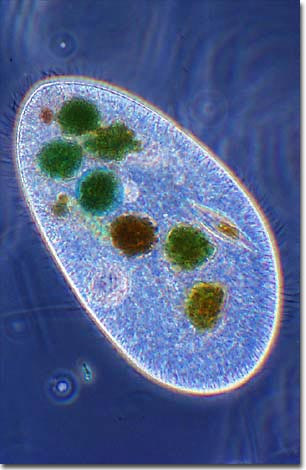This image presents a detailed close-up view of a microscopic single-cell organism, appearing under a microscope. The central organism is characterized by an oval shape, outlined by a glowing, almost rainbow-like border. The interior of the cell features several distinctive circular blobs, primarily green, but also includes one red and one yellow blob. These blobs vary slightly in hue and texture, adding complexity to the cell’s structure. Additionally, the cell contains subtle striations that diverge from the main circular areas, adding finer detail to the internal composition.

The setting around the cell is a predominantly blue field marked by wave-like and curved textures. This background also includes smaller dots and tiny organisms, one of which resembles an insect, positioned to the right, seemingly interacting with or within the cell. The entire scene has a vibrant glow, possibly an artifact from the microscopy process, highlighting the remarkable and complex features of this minute life form.